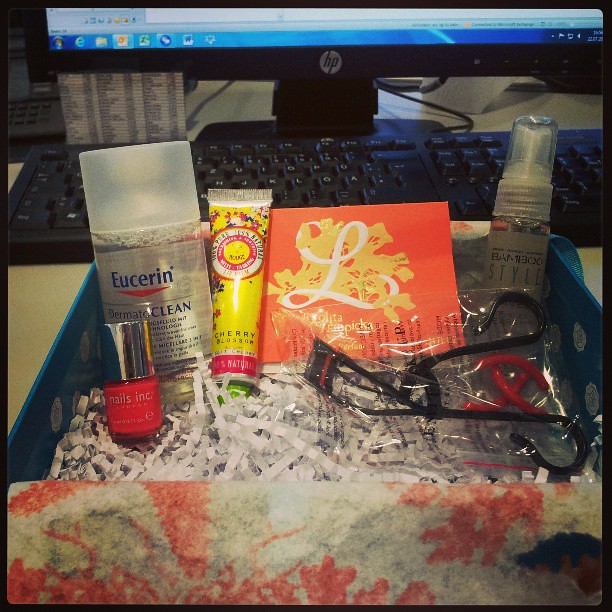The image features a cardboard gift box filled with various personal care items, nestled in white crinkle paper used as packing material. Among the items, there is a red 'Nails Inc' nail polish in a glass bottle, a large 'Eucerin Dermaclean' facial cleanser in a plastic container, a cherry blossom-scented all-natural lip balm in a small squeeze tube, an orange toothpick container with an 'L' on it, an eyelash curler still in its packaging, and a hair spritzer labeled 'Style'. The box and its contents are situated on a flat white desk. In the background, a black keyboard sits beneath a black HP monitor displaying the Windows taskbar with icons such as the start button, Internet Explorer, folder icons, and the time.